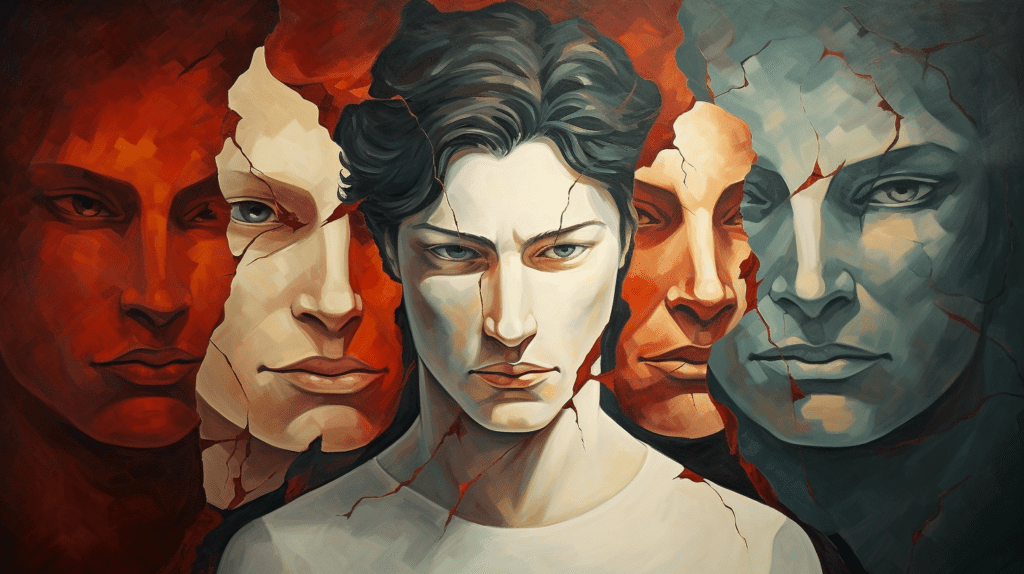This rectangular painting, wider than it is tall, centers on a close-up of a man from the upper chest up, wearing a white t-shirt. His short, wavy dark hair frames his porcelain-like, light skin, marked by bluish gray eyes that appear downcast. His angular face, featuring a prominent nose and jutting chin, is fractured as if wearing a cracked mask, revealing blood-like red splotches near his chin, left jawline, right shoulder, and along his forehead. His complexion remains consistent with bluish gray and pink accents, particularly noticeable on his cheeks. Surrounding the central figure are four iterations of his face, each depicted as fragmented masks in varied states. To his immediate left is a face devoid of hair, with red dominating its right side while the left side bears a crack extending through the cheekbone and eye. Further left, his entire face is bathed in red with no visible hair. To his immediate right, the duplicated face is smaller and exhibits more pronounced red cracks, with the cheek bearing more fragmentation and an orangish-red hue. The far-right rendition shows a gray and blue-hued face, with minor red cracks on the left cheek, extensive cracks across the forehead, and an absence of hair, replaced by grayish-blue tones that extend to the neck. Each repeated face varies slightly but is unified by the pervasive cracking motif and differing color palettes.